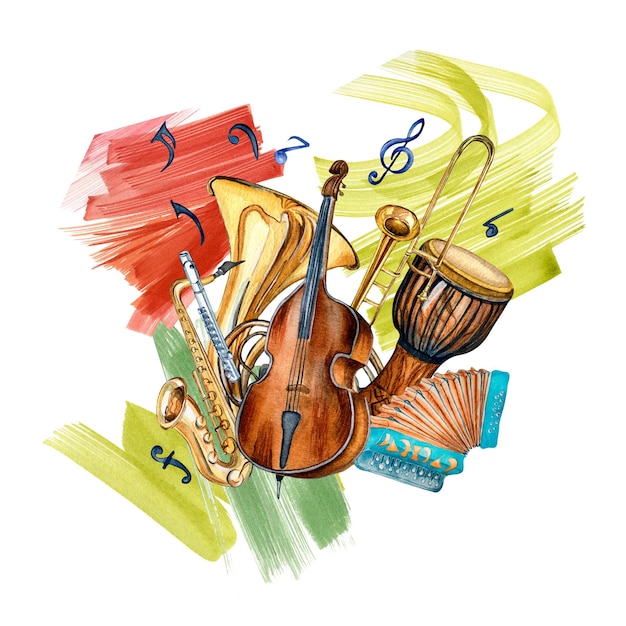This detailed drawing showcases a variety of musical instruments against a colorful background. In the foreground, the instruments stand out, featuring a violin, a bongo drum, a saxophone, a flute, a tuba, a cello, a trombone, and an accordion with a distinctive hot blue handle. The background is filled with dynamic, scraggly brushstrokes in vibrant shades of lime green, darker green, red, and rust, reminiscent of highlighter swipes. Interspersed among the vibrant colors are musical symbols, including the treble clef, some small notes, an F for forte, and the eighth note, all in dark blue. This piece combines the classic colors of the instruments with an energetic and colorful backdrop, creating a vivid and lively portrayal of musical elements.